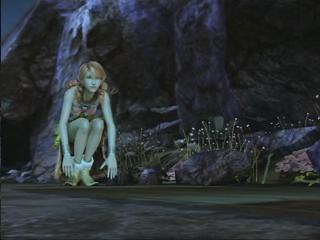The image captures an elf-like woman in a detailed fantasy gameplay setting. Her skin has a subtle, ethereal glow, and her hair, a vibrant mix of red and orange, cascades down as she crouches low to the ground. She is dressed in attire befitting her fantastical nature, including pointed shoes that hint at her swift agility. Behind her stands a prominent rock formation; its surface is predominantly gray with striking white accents, adding texture and depth to the scene. The ground in the foreground appears stone-like, with shadows adding a sense of realism and depth, and the surface carries a greenish tint. The background features dark gray stones interspersed with stray weeds and topped with white highlights, although the overall image quality retains a slight graininess. The scene exudes a mystical and somewhat desolate ambiance.